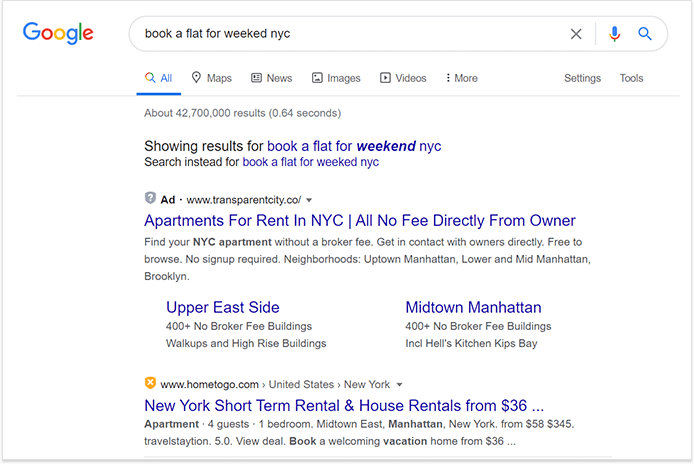**Caption:**

A screenshot of a Google search for "book a flat for weekend, New York City, NYC" shows the search results processed in 0.64 seconds with approximately 42,700,000 results. The interface displays the standard set of navigation buttons at the top: All, Maps, News, Images, Videos, More, Settings, and Tools. The search bar is prominently featured along with buttons for voice search and a magnifying glass icon for manual search.

The first search result is an ad listing apartments for rent in NYC, highlighting areas such as the Upper East Side and Midtown Manhattan. Detailed descriptions mention hundreds of available apartments with no broker fees and direct contact with owners. Specific neighborhoods mentioned include Hell's Kitchen and Kips Bay.

Scrolling further, the next result is not marked as an ad and discusses short-term rentals in New York, starting from what appears to be $36, though the price is truncated. The visible text provides a brief overview of various apartment options, like a one-bedroom in Midtown East Manhattan starting at $58, along with a mention of a vacation home listing with the Travel Station rating it highly at 5.0. The text and navigation elements are rendered in a typical Google search layout, ensuring a familiar and user-friendly experience.